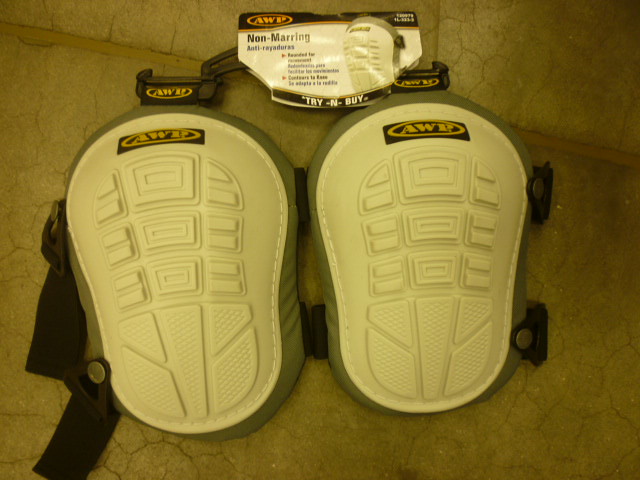This is a photograph of a pair of white, textured, molded plastic knee pads, designed to offer protection. The knee pads feature black fastening straps on each side, likely for securing them around the knees, and they rest on a green fabric surface. Above the knee pads, still attached to their packaging, is a paper label with a prominent black and gold triangular logo that reads "AWP" in stencil-style yellow letters. Additionally, the label reads "non-marring, anti-rigidourous, try before you buy," though parts of the text are blurred and hard to discern. The knee pads also have the AWP brand logo printed on them. Beneath this setup, the green fabric lies on a stone or concrete floor, which has noticeable cracks.